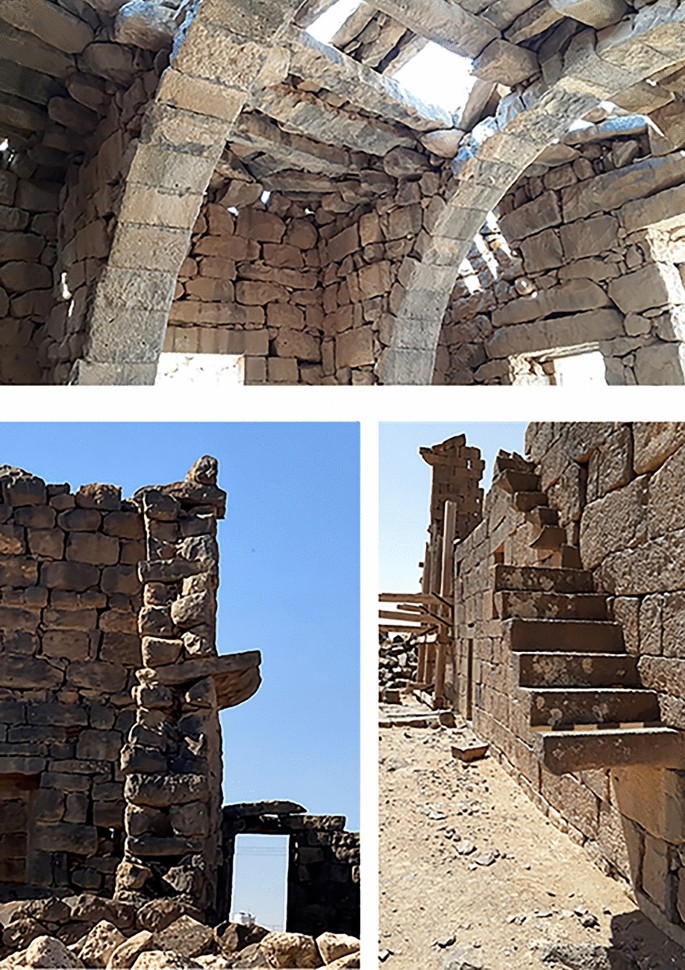This is a detailed collage of three photographs capturing various perspectives of an ancient stone building's ruins. The top 40% of the image showcases the interior of what appears to be a stone structure with two supporting cross archways. The arches, crafted from gray and light brown stones, frame partial views of holes that might have been doors or windows—the roof is largely absent, allowing sunlight to filter through the openings. The remaining 60% of the collage is split into two vertical photos. The bottom left photo presents the building's exterior corner against a backdrop of a clear blue sky, highlighting a tall stone façade with intricate designs that resemble a former chimney or architectural detail. The bottom right photo depicts an exterior wall with a dilapidated stairway comprising five or six steps, which are elevated above the ground and lead to nowhere, emphasizing the structure's disheveled condition. A mix of dirt and debris surrounds this area, further accentuating the ruinous state of the abandoned building.